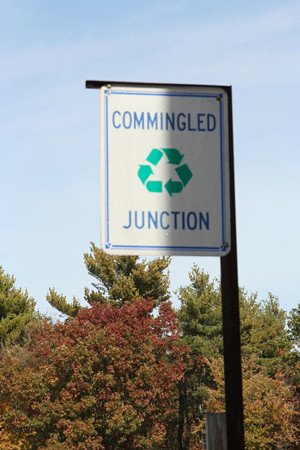The color photograph captures a street sign marked "Commingled Junction" with a blue border and a green recycling symbol at its center. Positioned on a pole near a street, the sign is partially shaded, casting shadows on its right side. Above, a clear blue sky with light white clouds frames the scene, while tall trees, some with reddish autumn leaves, create an inviting backdrop.